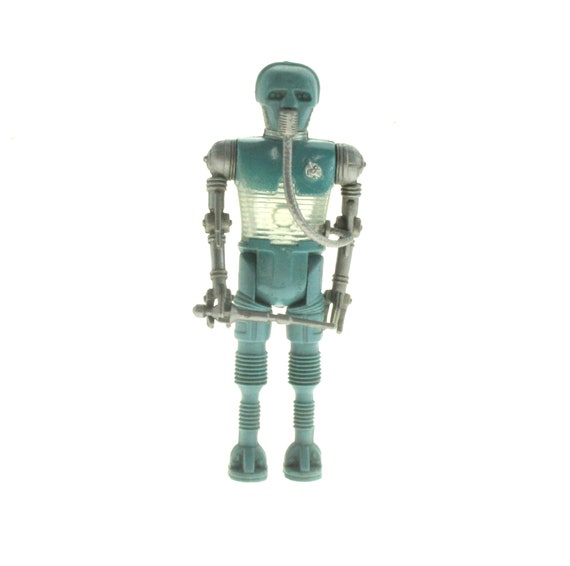This is a photo of a toy plastic robot, reminiscent of a 1960s design with a distinctly human look, standing upright against a plain white background. The robot's head is bluish-gray, and its torso is predominantly light blue with a clear plastic section in the chest area that appears to house a light. The robot's arms are gray and hang straight down, with the right hand holding a weapon that looks like a short sword or lightsaber. The robot also features a mask connected to an oxygen tube that runs from its mouth, wraps around its left arm, and connects to its back. The lower body, including the legs and round feet, is the same light blue as the mask and shoulders, and the feet resemble suction cups. The robot is constructed from various individual sections: head, torso, arms, and legs, creating a detailed and segmented appearance.